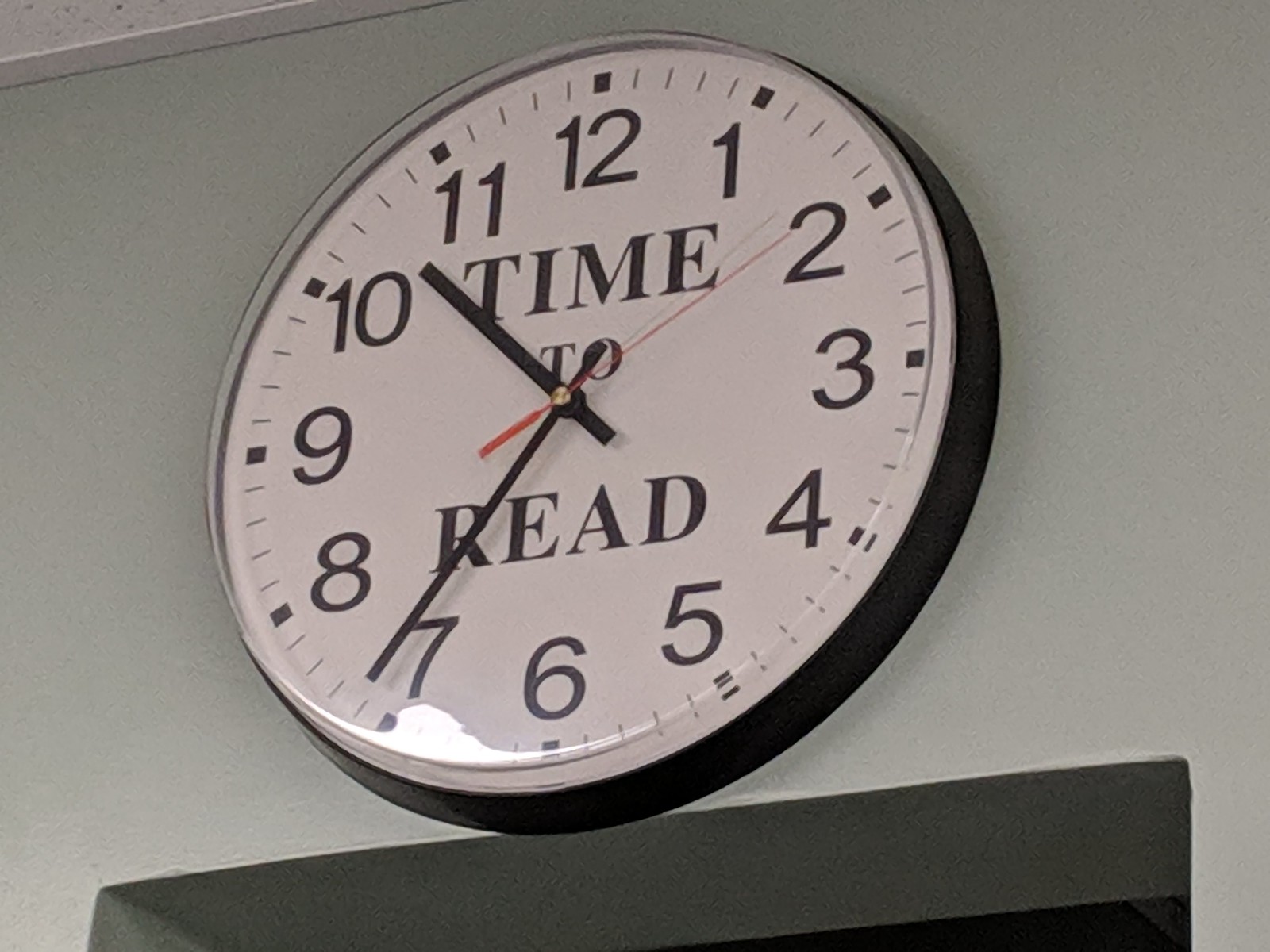This square photograph captures a wall-mounted clock set against a very light green background. The upper section of the image reveals a portion of the ceiling, which is white and speckled. Below the clock, there is the top part of a doorway, rectangular in shape, within which only darkness is visible. The clock features a black frame encasing a white face, with traditional black numbers for the hours and smaller notches marking the minutes. It also has black hour and minute hands, as well as a red second hand. A unique detail of the clock is the phrase "Time to Read" printed at its center. The time displayed is approximately 10:36 and 10 seconds. Overall, the clock has a minimalist design that emphasizes functionality and readability.